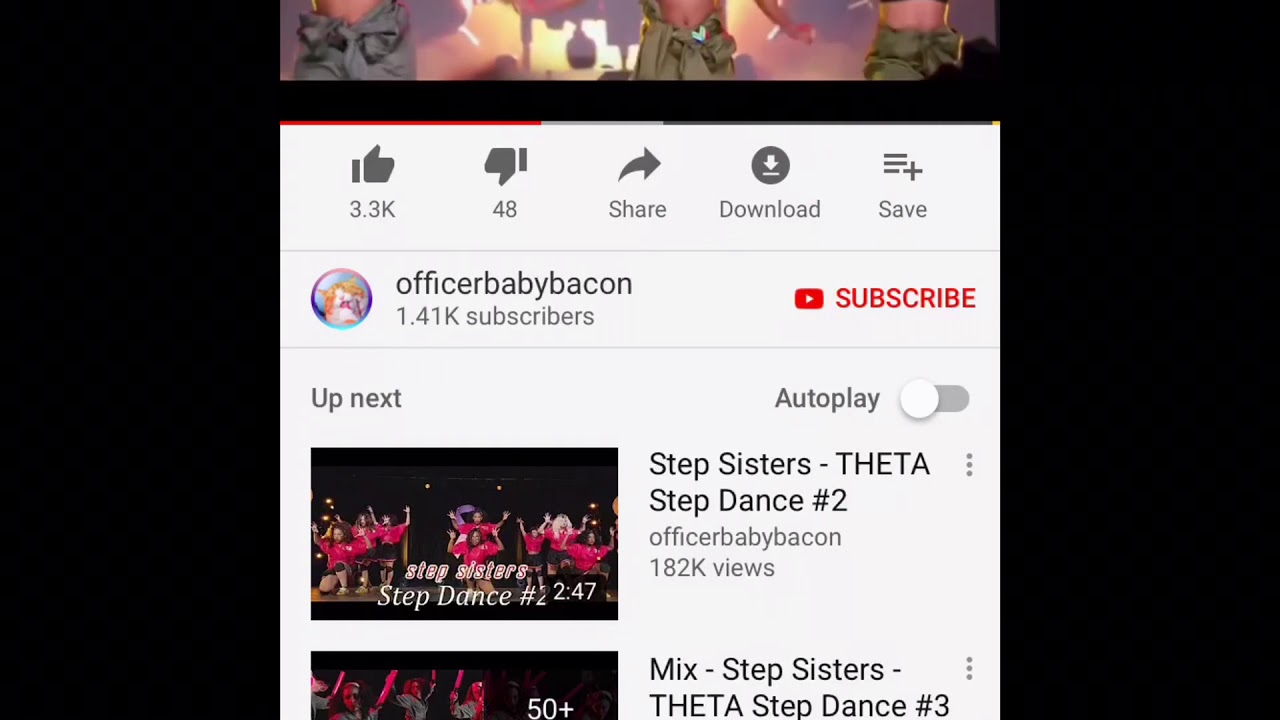The image appears to represent a digital interface, resembling a phone screenshot, though it is not one. The main focus is a central column flanked by two thick black bars on either side. At the very top, there is a cropped image of what seems to be three women, potentially performing on a stage; however, only their midsections (bellies and the tops of their pants) are visible.

Beneath this cropped image, the interface displays several interactive buttons: like, dislike, share, download, and save. Following these buttons is a user icon next to the username "Officer Baby Bacon," along with the subscriber count of "1.41k subscribers". To the right of this information is a prominent red subscription button labeled "Subscribe".

Continuing down the column, on the left side, the text "Up Next" is displayed. On the right side, aligned with "Up Next," is an "Autoplay" toggle button. Below this, there are thumbnails for upcoming videos. The first thumbnail, showing people dancing, is partially visible and labeled "Step Sisters Step Dance Number Two," though part of the name is obscured by a time bar displaying "2.47". Next to this, additional information shows the title "Step Sisters Theta Step Dance Number Two," the uploader's username, and "182k views." Beneath this, another partially visible thumbnail shows more people dancing with the text "50 plus," followed by the title "Mixed Step Sisters Theta Step Dance Number Three."

This detailed depiction encapsulates the structure and elements of the image, providing a comprehensive understanding of the visual content.